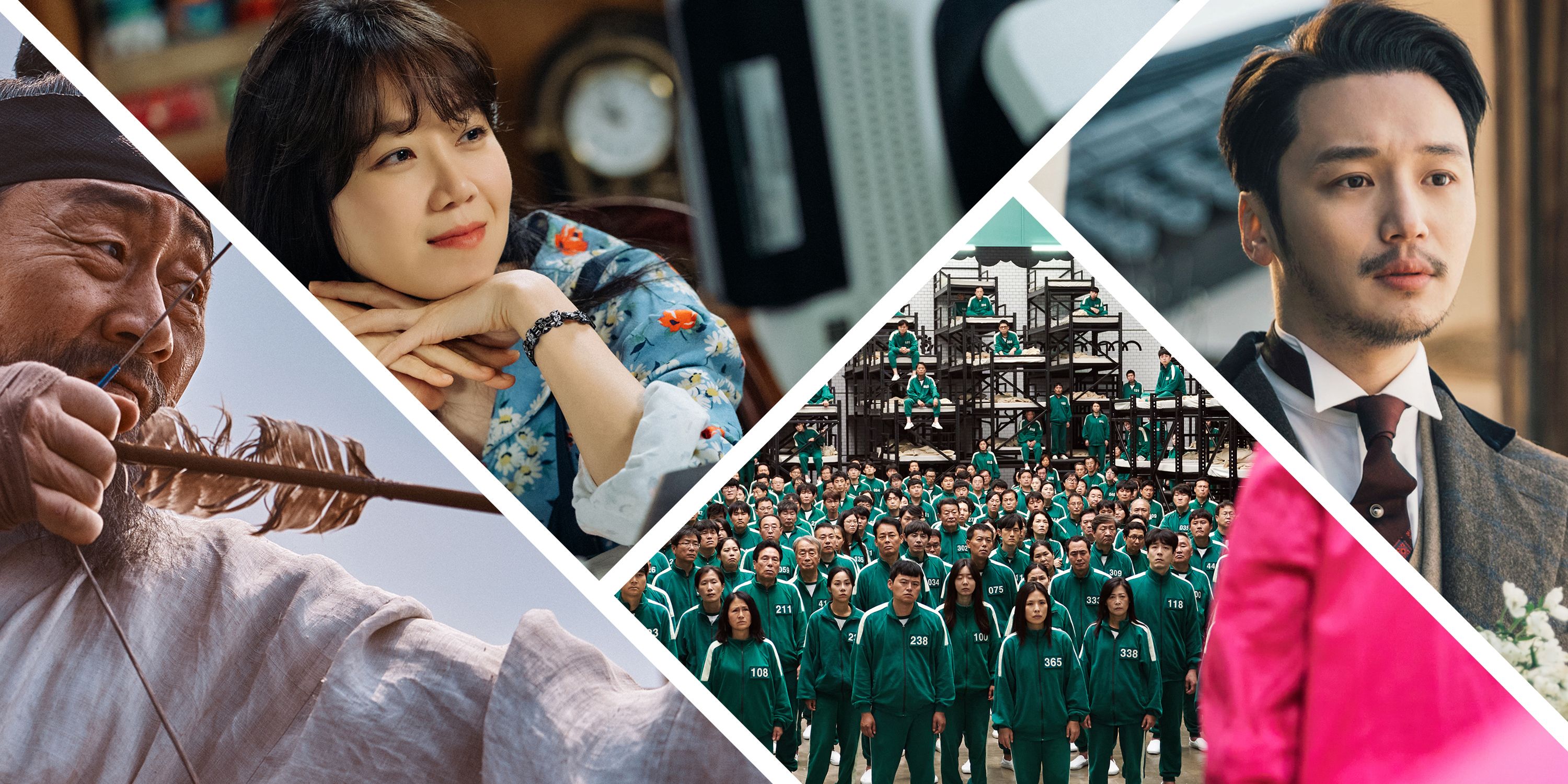This rectangular composite image features four distinct, irregularly-shaped photos of Asian individuals, artistically divided at various angles. On the far left, an older Asian man, wearing a black headband and a white long-sleeve shirt, is captured in the act of pulling back an arrow on a bow, with the arrow's tail and bowstring prominent in the frame. Adjacent to him, in an upside-down triangular section, a young Asian woman in a blue dress adorned with red and white flowers leans forward with her chin resting on her hands, dreamily gazing ahead. She wears a bracelet on her left wrist, and the blurred background shows a fancy grandfather clock, suggesting an interior setting. The top-right section, featuring a young Asian man with a beard and goatee, presents him in a gray suit with a maroon tie holding some flowers, also looking dreamily into the distance with a similarly blurred backdrop. In the bottom center, a larger geometric section portrays a group of Asian individuals in green tracksuits with numbers on their chests, reminiscent of a scene from the television show "Squid Game." A person in pink, potentially a guard from the show, stands addressing the group, with tall, scaffolded beds stacking up in the background.